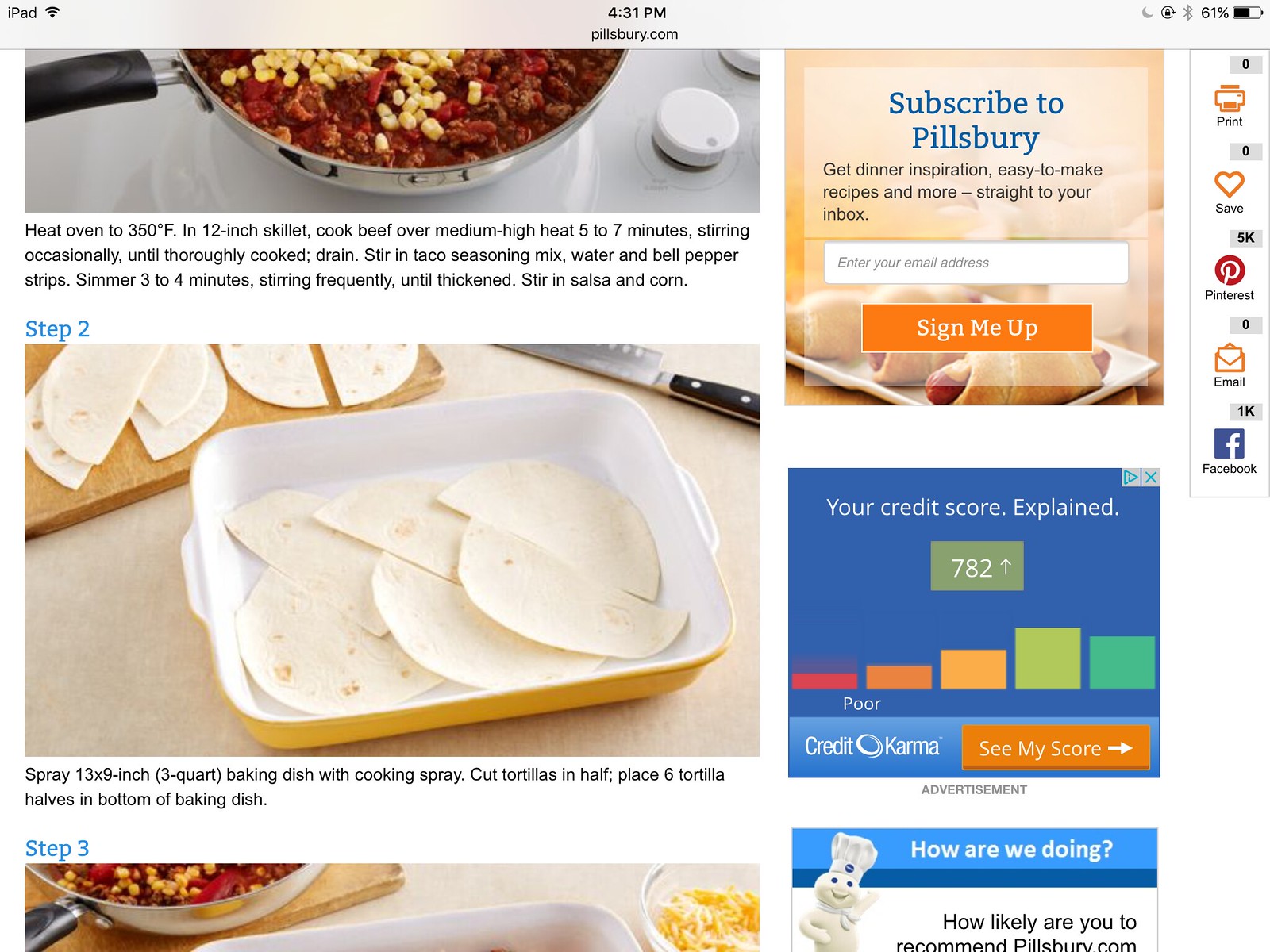The screenshot from an iPad displays a webpage from Pillsbury.com at 4:31 PM with 61% battery life remaining. The detailed image focuses on a step-by-step recipe. In the middle, a series of three color photographs shows different stages of preparation: a skillet pan simmering a red mixture of chili and corn on a stovetop, a yellow casserole dish containing six halved tortillas lined at the bottom, and finally, a partial glimpse of a cutting board with the casserole resting on it. Underneath these pictures, the step-by-step directions guide the cooking process, starting with heating the oven to 350°F and cooking beef with taco seasoning, water, and bell pepper strips, then adding salsa and corn.

On the right-hand side of the webpage, three advertisements appear in rectangular boxes. The top box invites users to subscribe to Pillsbury by entering their email, featuring blue lettering and an orange "sign me up" button. Below it, a Credit Karma ad with a blue background explains credit scores, displaying a sample score of 782 with colored bars representing various score ranges. The final box, in the lower right corner, shows the Pillsbury Doughboy logo and asks for user feedback with the prompt "How are we doing?" and "How likely are you to recommend Pillsbury.com?" Social media and utility icons for printing, saving, and sharing the page via Pinterest, email, or Facebook, are also present at the top right.